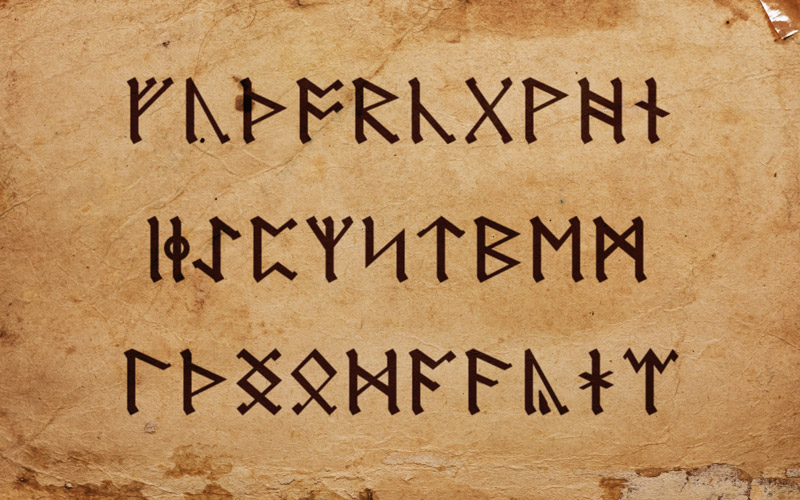The image depicts a rectangular photograph of ancient text written in what appears to be a runic or hieroglyphic script. The text consists of three lines, each containing approximately 10 characters, although the exact number is difficult to determine due to the interconnected letters. The letters are boldly written in dark brown or black ink on an old, beige-brown scroll or piece of paper that resembles worn cardboard. Notable features of the scroll include a folded top right corner and a faded bottom right section. The second line features a character resembling the letter 'M', and while some symbols may look familiar, many do not correlate to modern English. The text is centrally aligned on the paper.